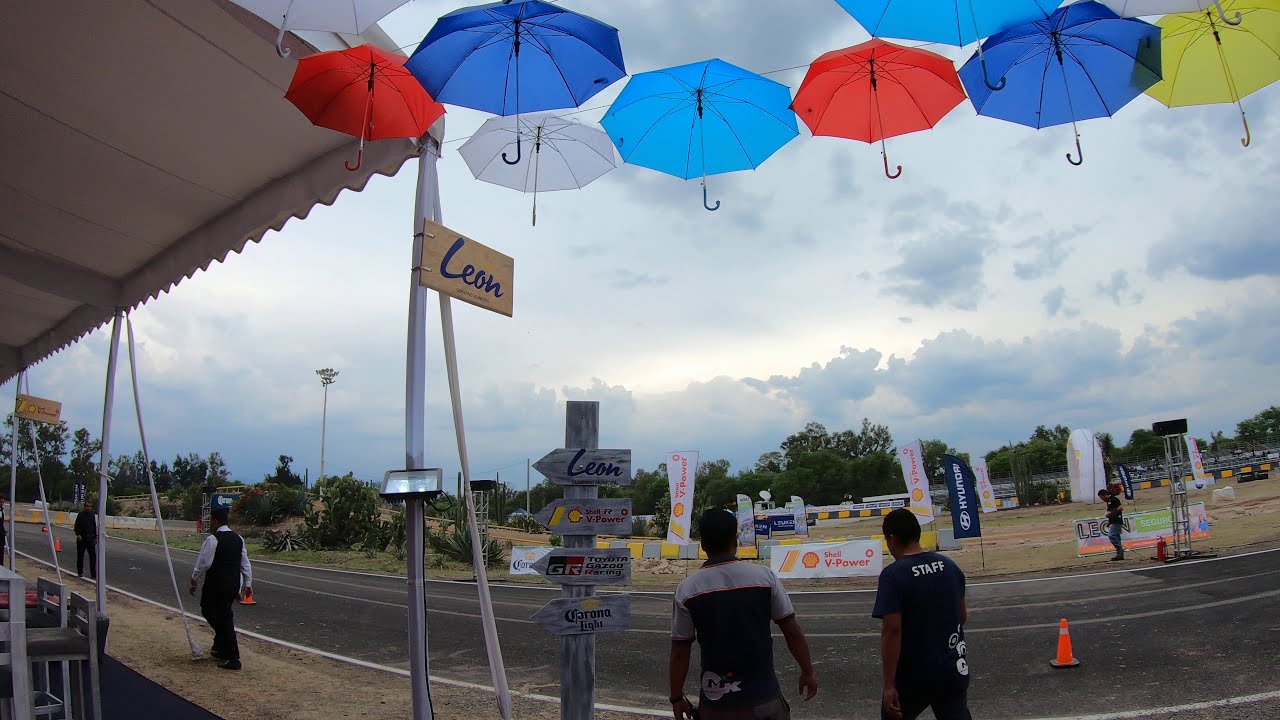In this outdoor scene, a cloudy sky with glimpses of sunlight peeking through serves as the backdrop. Suspended in the air are multicolored umbrellas – blue, red, yellow, and white – seemingly hanging from wires. Beneath these whimsical umbrellas, there is a curved racetrack lined with bright orange cones, suggesting a motorbike race rather than cars due to the track's size. 

In the foreground, two men with their backs to the camera appear to be working or preparing for the event. To their right, a solitary orange cone marks their position before the track begins. Off to the left, an awning supported by poles shelters a few more workers, who are also facing away. 

The background is dotted with an array of signs advertising brands like Corona Light, Toyota Racing, Shell V-Power, Hyundai, and Leon. The central area beyond the racetrack features more people, a dirt field, and green trees at the horizon. A sign attached to a canopy reads "Leon," indicating sponsorship or a promotional display.